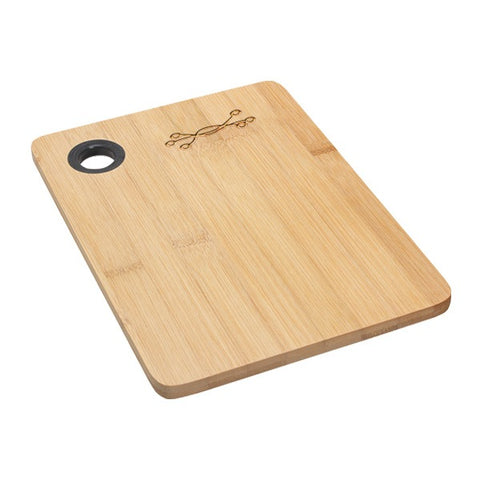This image depicts a light-colored rectangular wooden cutting board with rounded edges on an all-white background. Viewed from a roughly 45-degree top-down angle, the board is made of glued strips of cut bamboo displaying visible wood grain. In the upper left corner, there is a small round hole featuring a black insert made of either rubber, plastic, or another material, likely to prevent wear or facilitate hanging. Adjacent to the hole, a simple yet elegant carved logo consists of three intertwined curving lines, each ending in a small circle.